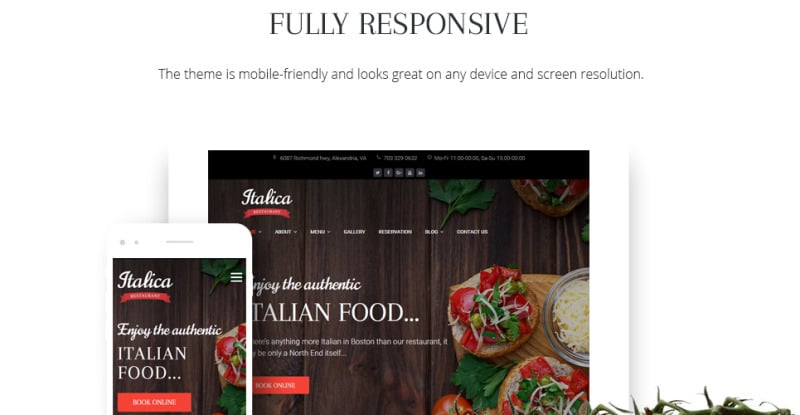This is a detailed caption for the given image:

---

The horizontal screenshot lacks upper and right-hand side borders and prominently features large grey text at the top center that reads, "Fully Responsive." Beneath this, a single line of smaller grey text explains, "The theme is mobile friendly and looks great on any device and screen resolution."

The main section of the image showcases both a tablet and a mobile phone. The tablet is positioned horizontally and overlaps with the top-left area of an adjacent mobile phone. Displayed on the devices are both the desktop and mobile versions of a website for a restaurant called "Italica."

In both the mobile and tablet views, the text "Enjoy the authentic Italian food" is visible under the restaurant's name. Further down, some text on the website version, partially obscured, reads, "anything more than Italian in Boston than our restaurant, North End itself," indicating that this is a Boston-based restaurant. 

A prominent red "Book Online" button is also shown, suggesting a call to action. The website's top menu bar—displayed on the tablet—features options labeled "About," "Menu," "Gallery," "Blog," and "Contact Us." 

The image also includes visual elements of presented Italian cuisine, depicting dishes with red, white, and green colors. Overlaid on the bottom right corner of the tablet are the stems of tomatoes, adding an authentic touch to the culinary theme.

---